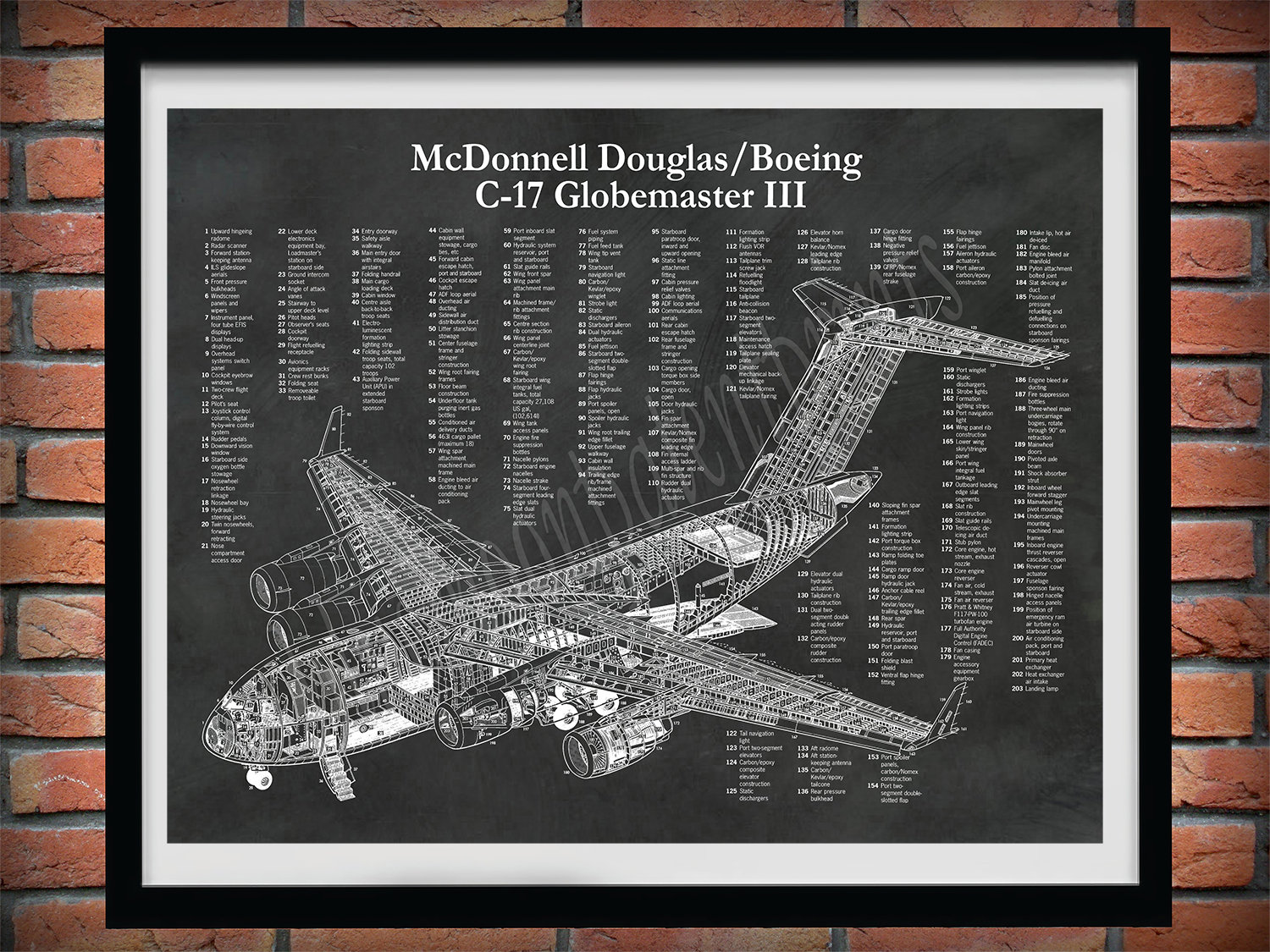This is a photograph of a framed poster hanging on a brick wall, featuring a comprehensive, detailed diagram of a McDonnell Douglas/Boeing C-17 Globemaster III airplane. The title at the top of the poster reads "McDonnell Douglas/Boeing C-17 Globemaster III" with the Roman numeral III properly denoting the third iteration. The poster, which has a white matting within a black frame, employs a black-and-white color scheme. The airplane diagram is drawn in a grid-style, reminiscent of a technical blueprint, displaying a transparent, see-through view of the aircraft's components, including the cockpit, four jet engines, and the expansive wings and tail. Numbers from 1 to 202 label each part of the airplane, which are meticulously detailed and explained in the surrounding columns of text. Each numerical label correlates with descriptions next to it, outlining the extensive and intricate parts required to construct the C-17 Globemaster III. The black backdrop contrasts sharply with the white text and diagrams, enhancing the visibility of the detailed technical illustrations and annotations.